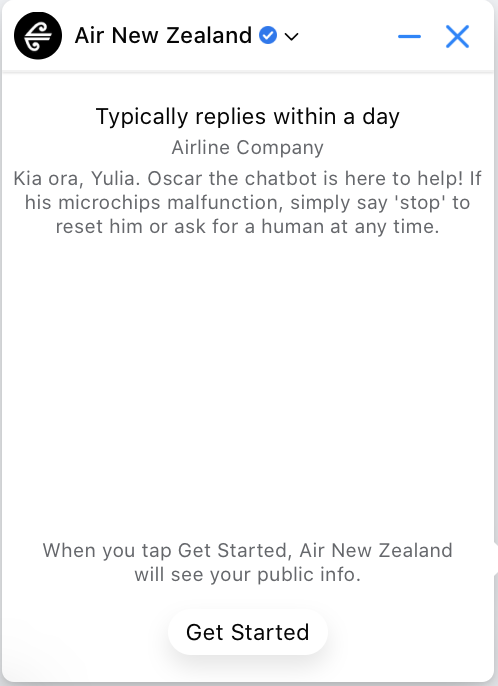The image depicts an app interface for Air New Zealand, featuring a technical support chat system. A central message informs users that the typical response time is within a day. The introduction introduces Oscar, the chatbot, who is available to assist users. If Oscar's microchips malfunction, users are advised to either reset him by saying "stop" or request to speak with a human agent at any time. At the bottom of the interface, a clickable button labeled "Get Started" allows users to initiate a chat session with the virtual assistant, presumably providing support related to Air New Zealand's services.